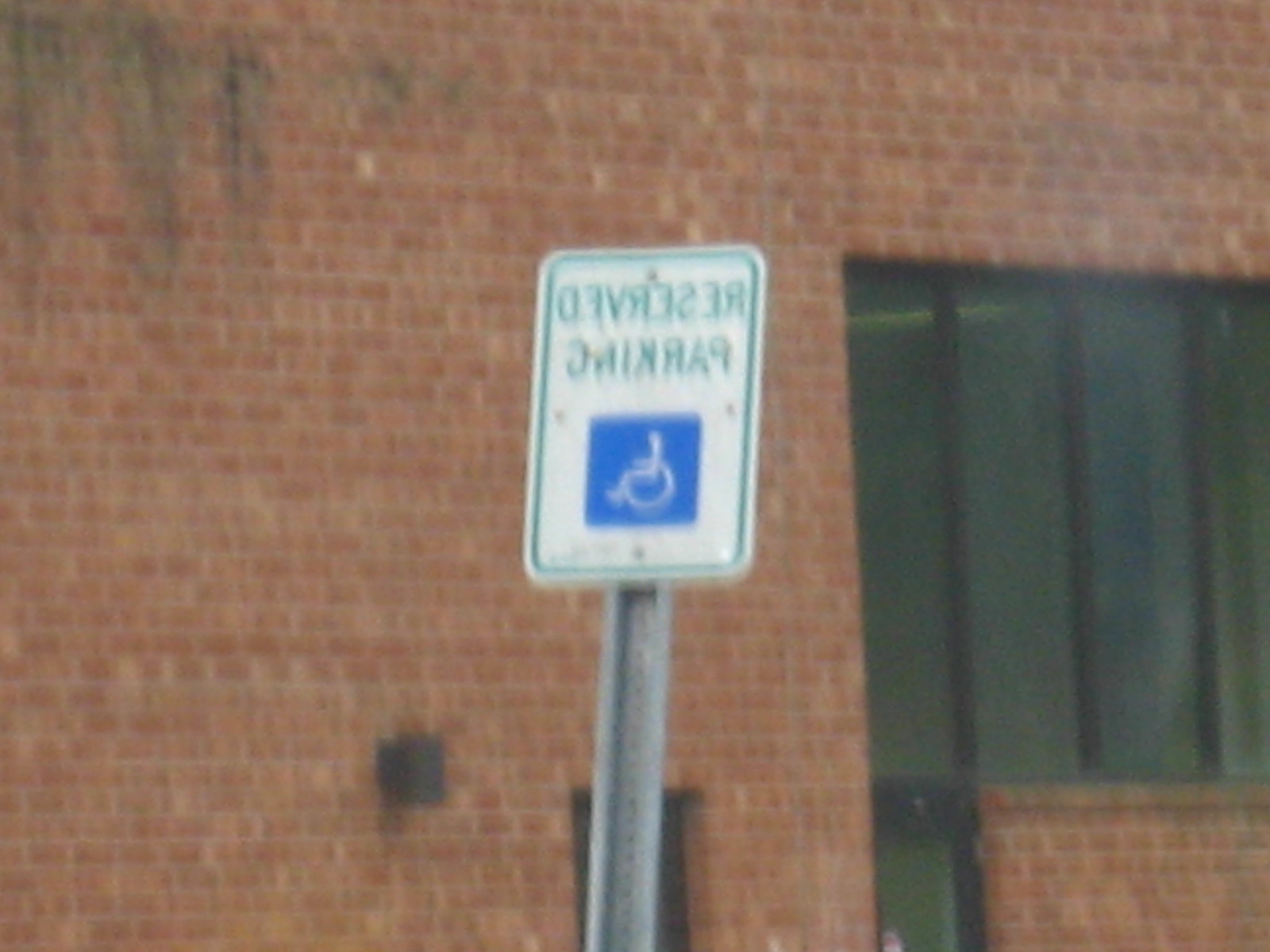This daytime photograph features the side of a red brick building situated on the right. The building displays multiple windows and possibly a doorway, partially visible. In the center of the image, a metal pole prominently holds a "Reserved Parking" sign, designated for handicapped individuals. The sign itself is white, with green lettering and a blue handicapped symbol. The overall setting is an outdoor parking area, with the sign clearly indicating designated handicapped parking adjacent to the building.